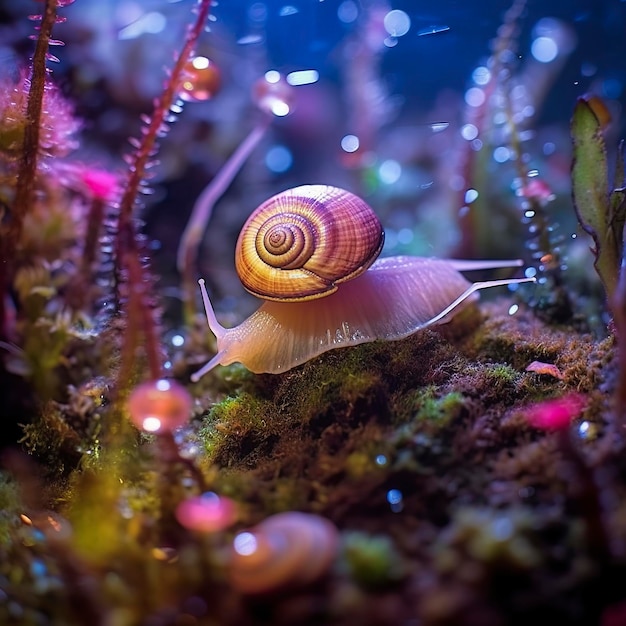This digital photograph captures a surreal, fantasy-like scene featuring a large, nearly translucent white snail. The snail, which is much larger than its small brown and orange shell perched on its back, is positioned at the center of the image, moving from right to left. It has two prominent antennae at the front and two similar appendages at the back, mimicking antennae. The snail is on a piece of artificial moss inside what appears to be an aquarium tank, adorned with various fake plants. The colors in the image are primarily greens and browns, interspersed with purples, yellows, blues, and whites, contributing to the photo's mystical atmosphere. Reflective lights create a bubble-like effect on the glass, adding to the image's dreamy quality. This combination of elements gives the photograph an edited, fantastical appearance, complete with a whimsical feeling.